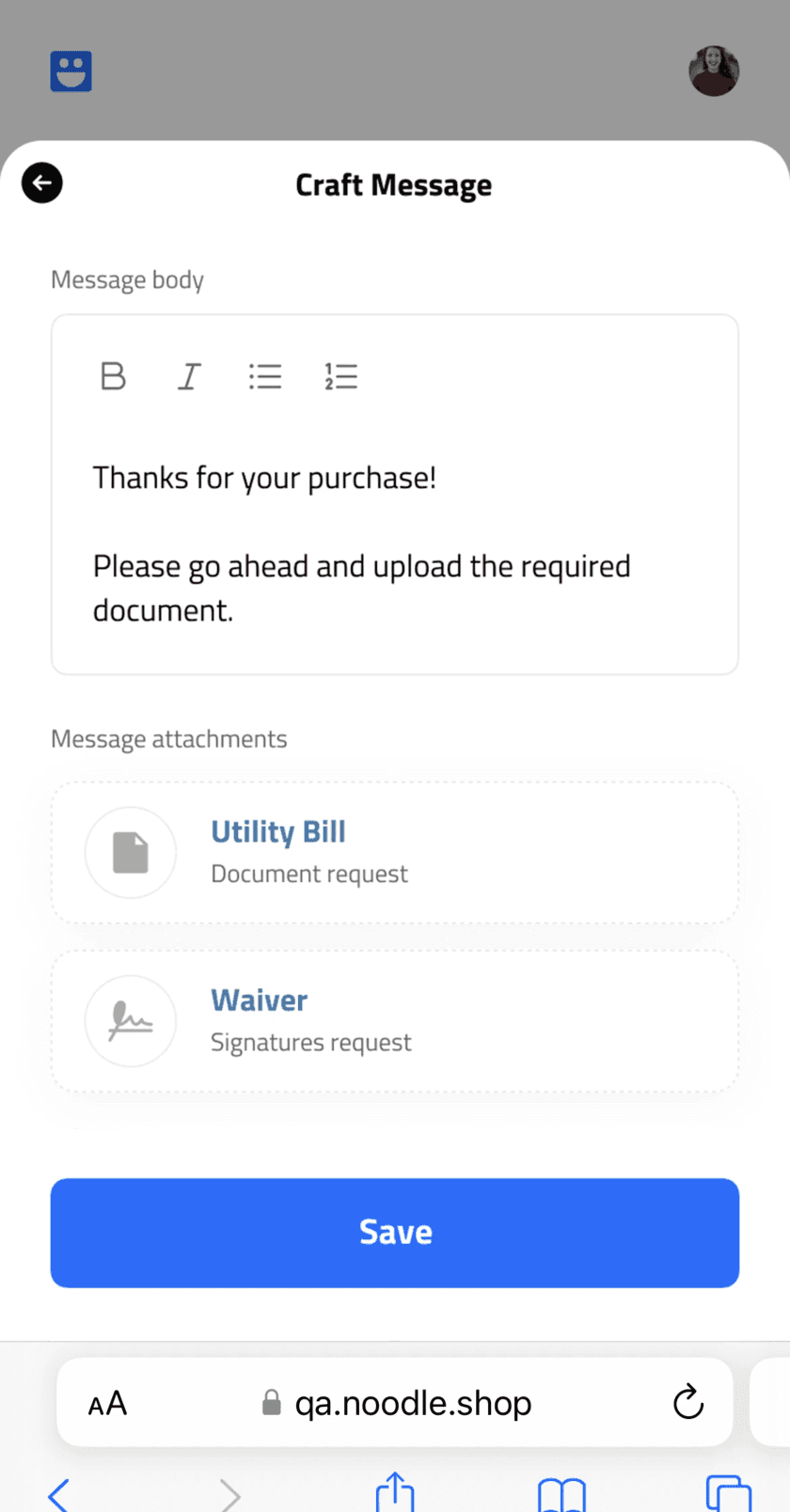A digital notification, possibly generated by AI, showcases a structured template for crafting messages. The top of the screen displays the heading "Craft Message" in bold black font. Below it is a text box labeled "Message Body," where users can type their messages. The template offers various formatting options, including bold, italics, and bullet points, to emphasize different parts of the message.

In this particular instance, the crafted message reads: "Thanks for your purchase. Please go ahead and upload the required document." Following the message, there is a section titled "Message Attachments," which lists two required documents: "Utility Bill" and "Waiver."

This setup implies that a business transaction is incomplete due to missing documents. The recipient, who has made a purchase from the business, is now requested to provide the necessary documents to finalize the transaction.

At the bottom of the screen, there is a blue "Save" button with white font, along with a website search bar displaying the URL "qa.noodle.shop." This indicates that the message is part of a larger user interface, likely a customer service platform or communication tool.